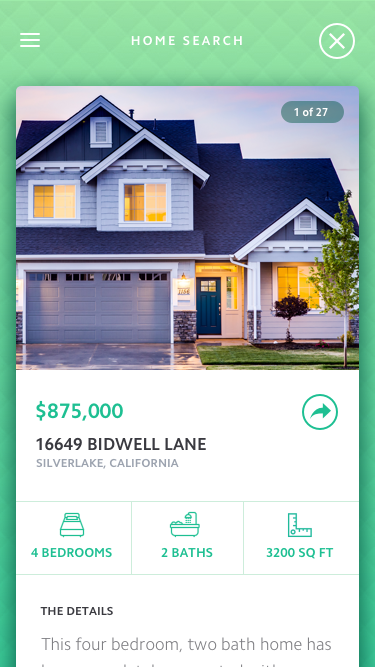The background of this image is a bold green, featuring an intricate pattern of green diamonds. At the center, prominent white text reads "Home Search," with a white circle containing an X to the right of the text. The main focus of the image is a beautifully designed blue house. The house boasts a blue garage, a cozy porch area supported by a white column, and a dark blue front door. The exterior siding is a lighter blue, and the windows emit a warm yellow glow.

At the top of the image, the text reads "1 of 27," indicating that this is the first of 27 pictures. Below this, the house's price is listed at $875,000. The address, displayed in uppercase, is 16649 BIDWELL LANE. Situated in Silver Lake, California, the location details provide additional context.

On the left side, green icons and text indicate the home’s features: four bedrooms (accompanied by an image of a bed), two bathrooms (illustrated with a bathtub icon), and a total area of 3,200 square feet (highlighted by a ruler icon).

Finally, at the bottom, black text introduces "The Details," followed by lighter black text that begins to describe the property: "This 4 Bedroom 2 Bath Home Has..." The information ends abruptly, leaving the description incomplete.